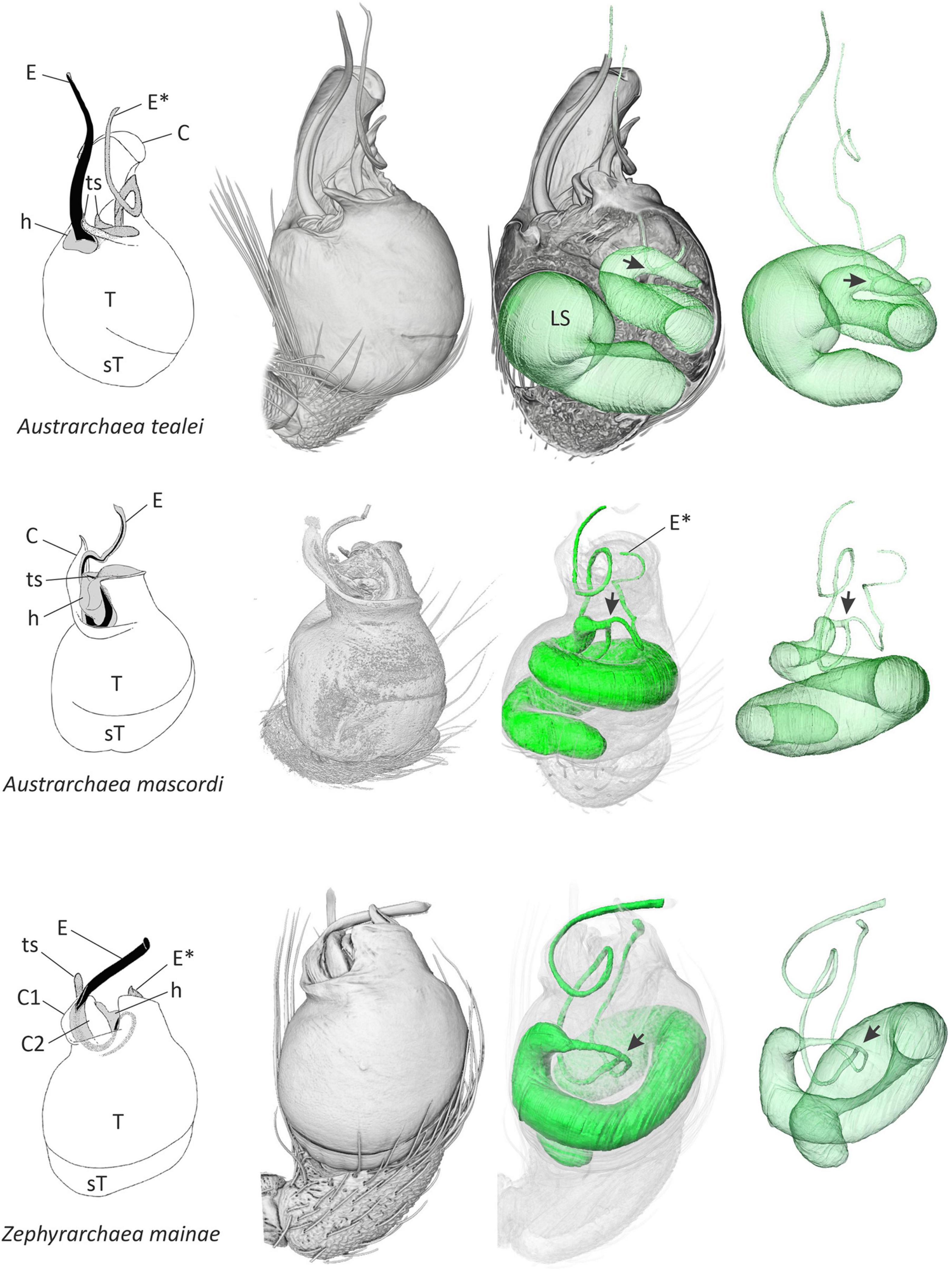This scientific poster illustrates detailed anatomical diagrams of various biological organs, specifically the heart-like structures of different spider species. Down the left side of the poster, there are black-and-white line renderings of these organs labeled with scientific names and identifying letters pointing to specific parts. Each spider species is represented in rows, depicting four progressive images. 

The first row features Austroarchaea telei, starting with a clear line drawing labeled with call-outs such as S-T-T-H-T-S-C-E. The second row is for Austroarchaea maschordii, similarly starting with a labeled line drawing. The third row showcases Zephyrarchaea manii in the same manner. 

Each row includes four images: the first one is a labeled line drawing, the second shows the same organ with gray shading, highlighting detailed structures within the organ. The third image displays the organ sectioned to reveal a green-highlighted internal structure, which at first appears as two irregular masses but is clarified in the final image. Here, the external organ is removed, leaving only the green internal structure, demonstrating a clearer view of the internal pieces without the outer layers. 

These meticulously detailed images show the progression from the exterior to the interior anatomical features, emphasizing the intricate structure of these spider organs, akin to the layout of a textbook illustration.